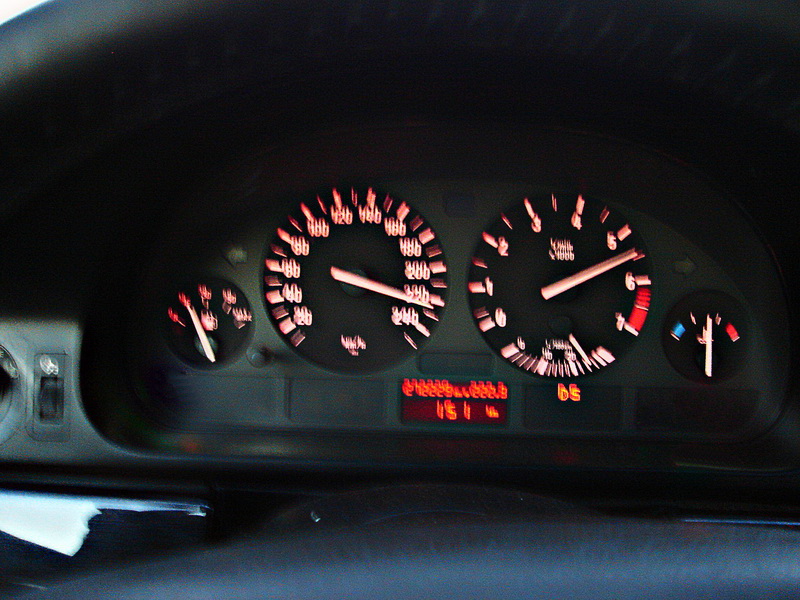This image captures an inside view of a vehicle’s dashboard, slightly blurred due to motion. The instrument panel is framed by a black background, and the top edge of the steering wheel is partially visible at the bottom. 

On the left side of the dashboard, the image shows a partially visible semicircle, the purpose of which is unclear. Adjacent to it is a black, rectangular component that resembles a roll track, bearing a white symbol that is too blurred to decipher.

Dominating the dashboard are four circular gauges. The two outermost circles are smaller than the two central ones. The far-left circle is a fuel gauge with a white needle pointing to the second mark from the left, suggesting the fuel level is low. The symbol for the gas tank is also visible, along with five calibration marks.

The first large central circle is the speedometer, with white numerals and increments marked at 20, 40, 60, 80, 100, 120, 140, 160, 180, 200, 220, and 240. The speedometer needle points to about 228. 

The second large circle is a tachometer, also with white numerals ranging from 0 to 7, where the area between 6 and 7 is highlighted in red. The needle is reading approximately 5.5.

The far-right small circle has a white needle pointing straight up, indicating a medium value. The gauge has four calibration marks, with the leftmost marked in blue and the rightmost in red, suggesting it monitors temperature. 

Below these circles, a rectangular digital screen likely serves as the odometer, although the numbers are too blurred to discern. To its right is another rectangular section displaying orange letters, which seem to spell "DS."